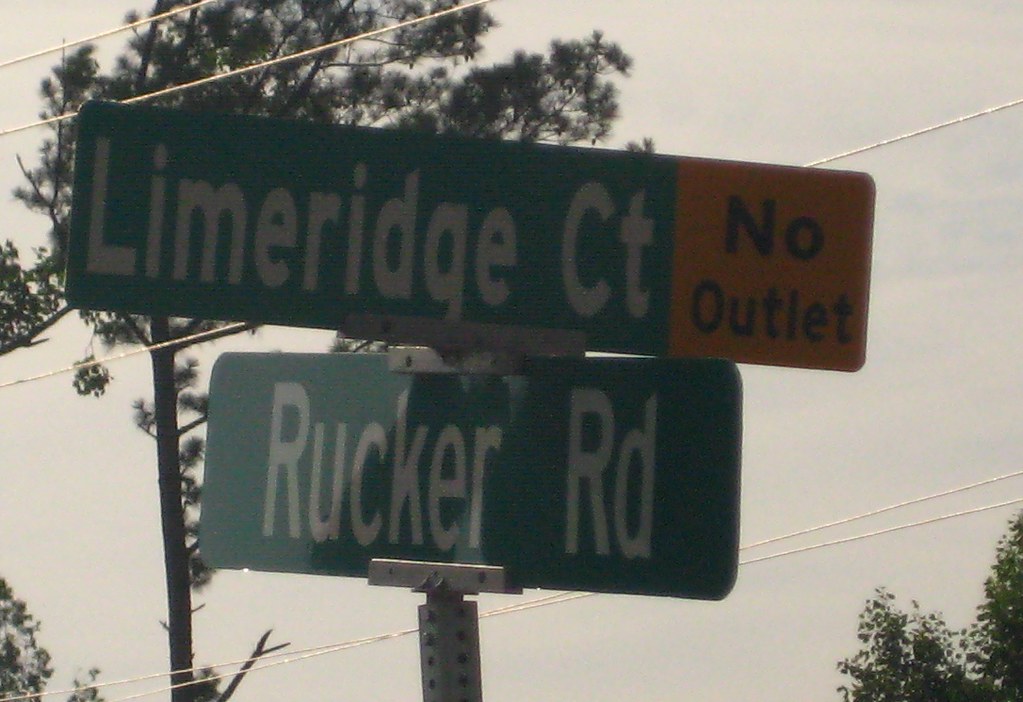This photograph prominently features a pair of street signs against an overcast sky. The signs, mounted on a steel-colored pole, indicate the intersection of Limber Ridge Court and Rucker Road. The street names are displayed on the familiar green metal backdrop, typical of most road signs found on interstate highways. Notably, the sign for Limber Ridge Court also includes a yellow "No Outlet" warning. In the background, the sky is predominantly cloudy, creating a muted, grayish atmosphere. Various trees are scattered throughout the scene, with a few tall trees visible in the distance and a smaller tree occupying the bottom right corner of the image. Additionally, power lines are faintly visible, stretching across the sky in the background.